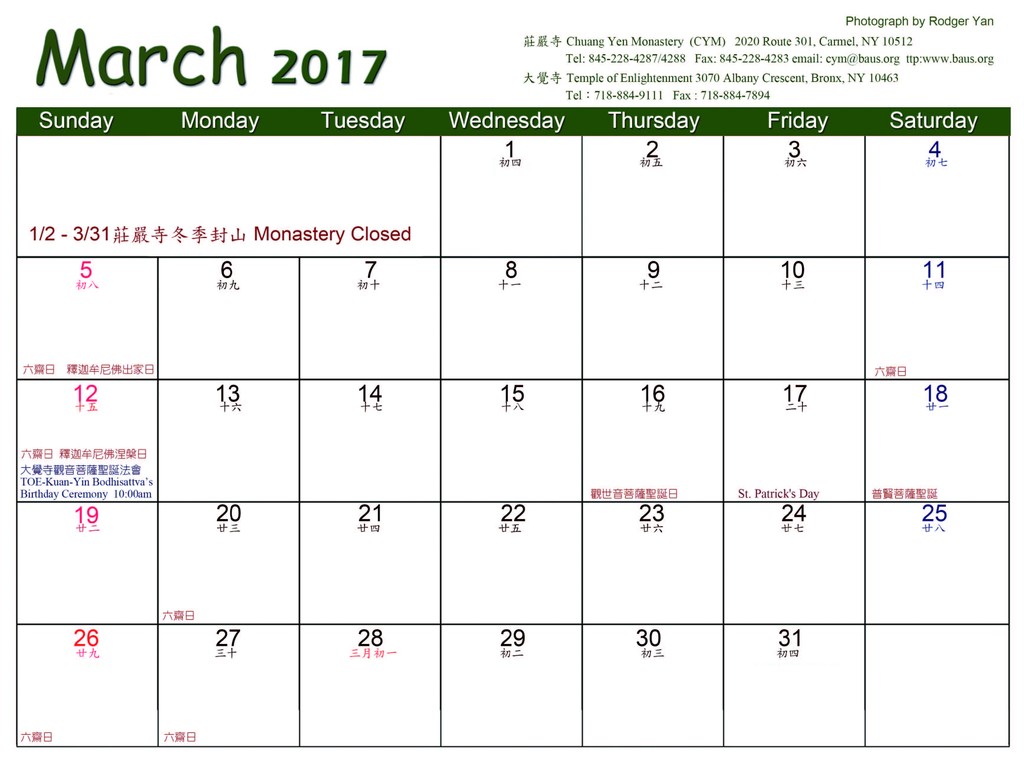This image depicts a detailed calendar page for March 2017, with both English and Asian language elements. The title "March 2017" is prominently written in dark green letters at the top. Below it, a slim green rectangle spans the width of the page, listing the days of the week: Sunday through Saturday. Each Sunday is marked with red numerals, while weekdays are marked in black, and Saturdays in dark blue.

The left top part of the calendar includes Asian characters translated into English, indicating "Monastery closed," with details spanning from the 1st to the 3rd and the 31st. The calendar features a bilingual layout with annotations written in both an unspecified Asian language and English. Notable English annotations include "St. Patrick's Day" observed on the 17th and various other entries that mark significant events, such as March 5th, 12th, 16th, 18th, 20th, 26th, and 27th, though not all details are readable. Additionally, the photograph credit "Photographed by Roger Yan" is included, along with references to "Chuang Yen Monastery," its address in Carmel, New York, and the "Temple of Enlightenment" in the Bronx, New York. Special mention is made of "Chuang Yen’s 10th birthday ceremony" scheduled at 10 a.m. on an unspecified date.